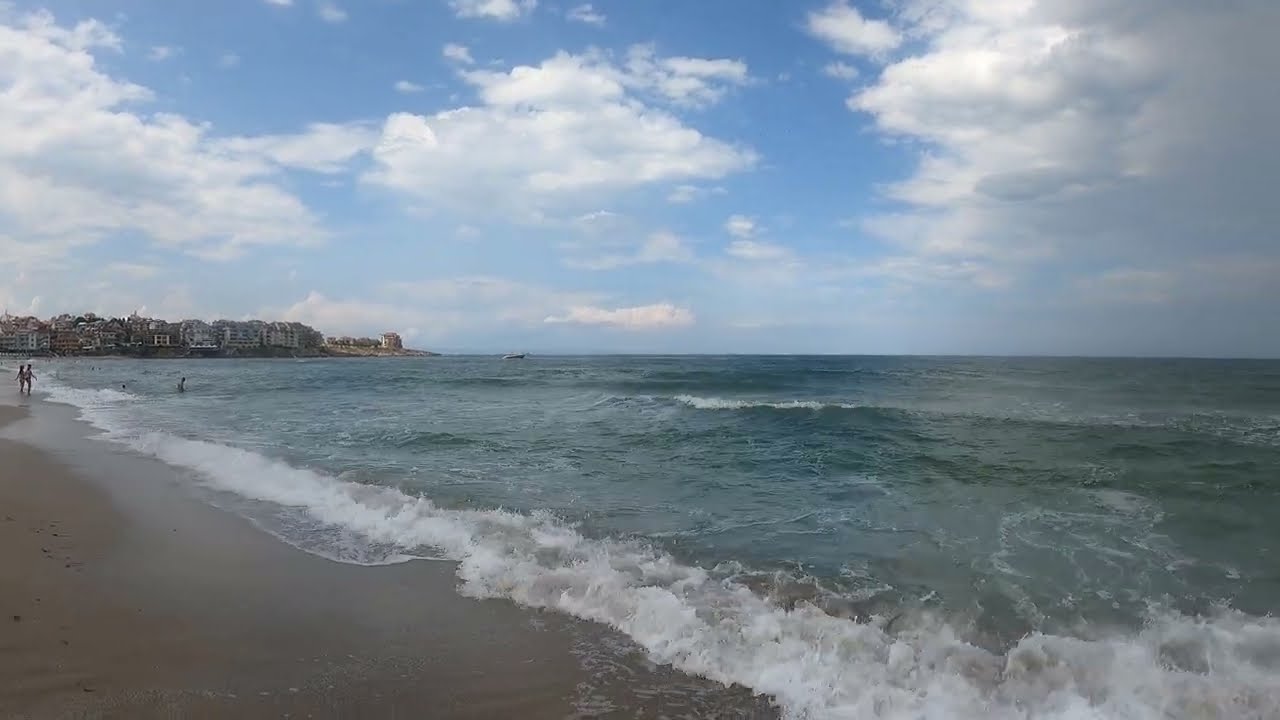The image depicts a wide, rectangular scene of an ocean shoreline on a slightly overcast day. The horizon line splits the image horizontally, with a bright blue sky adorned with several thick, puffy white clouds casting shadows over the deep greenish-blue sea. In the distance, on the left side of the horizon, a cluster of buildings, likely hotels, condos, or beachfront properties, can be seen on a landmass extending into the water. The left corner of the image reveals a stretch of wet, grayish sand with a couple of people standing near the edge of the water, where white foamy waves diagonally meet the coast. Further off in the distance, there is a boat anchored just offshore, and a few people are seen walking along the lightly shaded sand or swimming in the surf. The overall ambiance suggests a cool, slightly shady day with no harsh sunlight but sufficient daylight to illuminate the serene coastal scene.